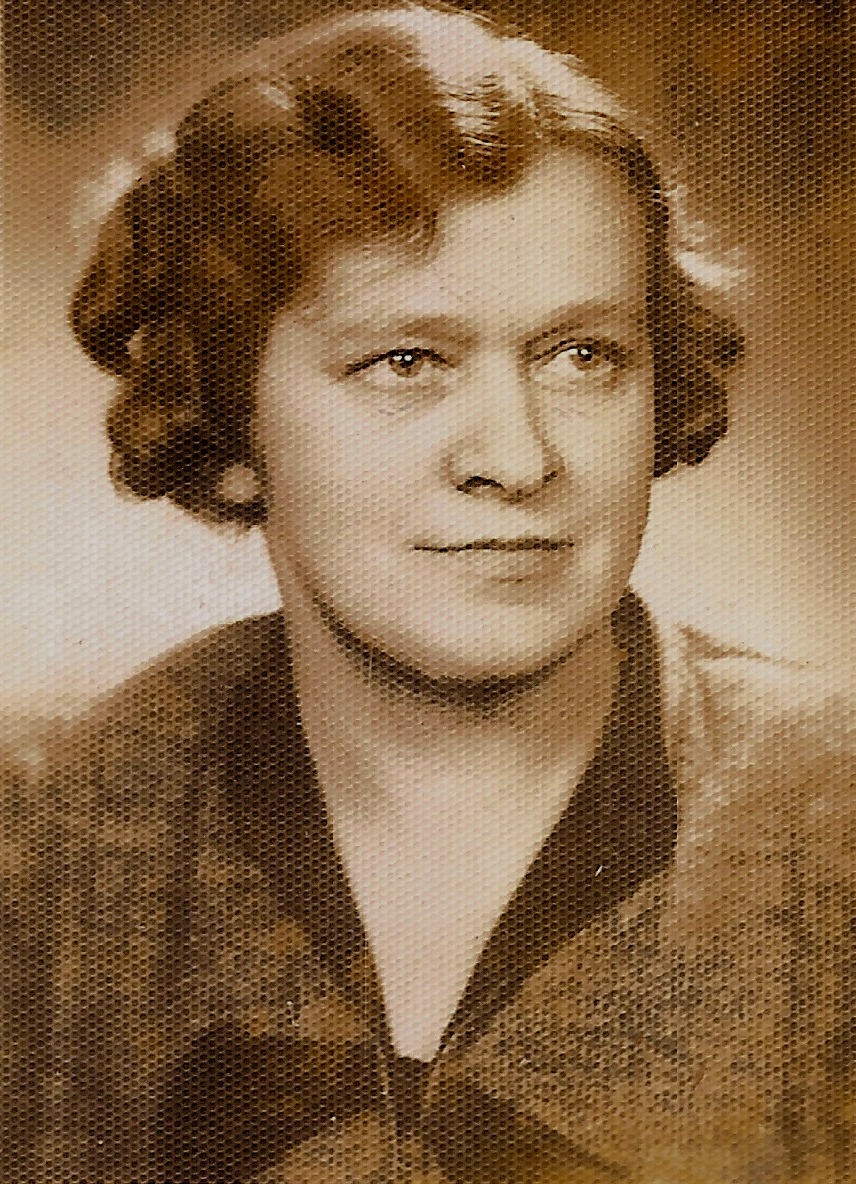The portrait is a sepia-toned photograph of a young woman, likely taken between the 1920s and 1950s. The image, which has a grainy texture, appears to be professionally done, reminiscent of old-fashioned studio photography. The woman, possibly in her 20s or 30s but dressed conservatively enough to look older, gazes off into the distance with a subtle, almost imperceptible smile. Her short, wavy hair, styled just below her ears, frames her face and is gently illuminated by classic portrait lighting. She wears a blouse with a collar, extending to her breastbone, and no visible jewelry or heavy makeup, further contributing to her understated appearance. The background features a gradient from dark to light, enhancing the nostalgic quality of the scene.